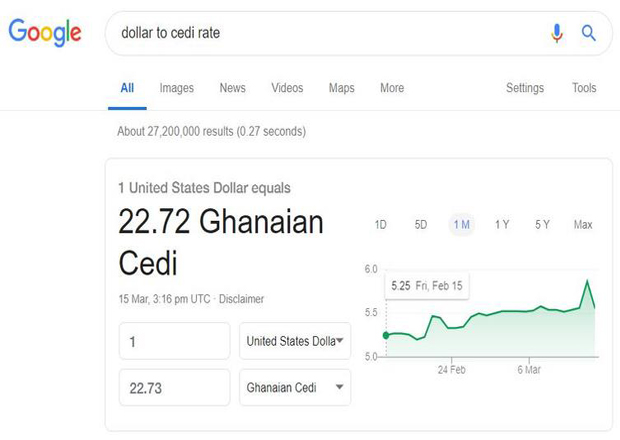Screenshot of a Google search result for currency conversion: The search query "dollar to Cedi rate" is entered in small black text within the search bar. Below this bar are tabs for different types of search results, labeled from left to right as All, Images, News, Videos, Maps, More, with Settings and Tools on the far right. The "All" tab is highlighted with a blue underline, indicating it is the selected category.

Directly underneath these tabs, in black and gray text, it is displayed that one United States Dollar is equivalent to 22.72 Ghanaian Cedi. Further down, there are fields and buttons allowing users to convert different amounts of currencies, defaulting to 1 USD to 22.73 GHS. To the right of this conversion information, a line graph with a green line shows the historical exchange rate trend of these currencies over time.

The Google logo, in its trademark colorful letters, appears at the top left of the webpage. The entire page is set against a plain white background, with most text in small, standard font, and colored in a dark gray or black hue.